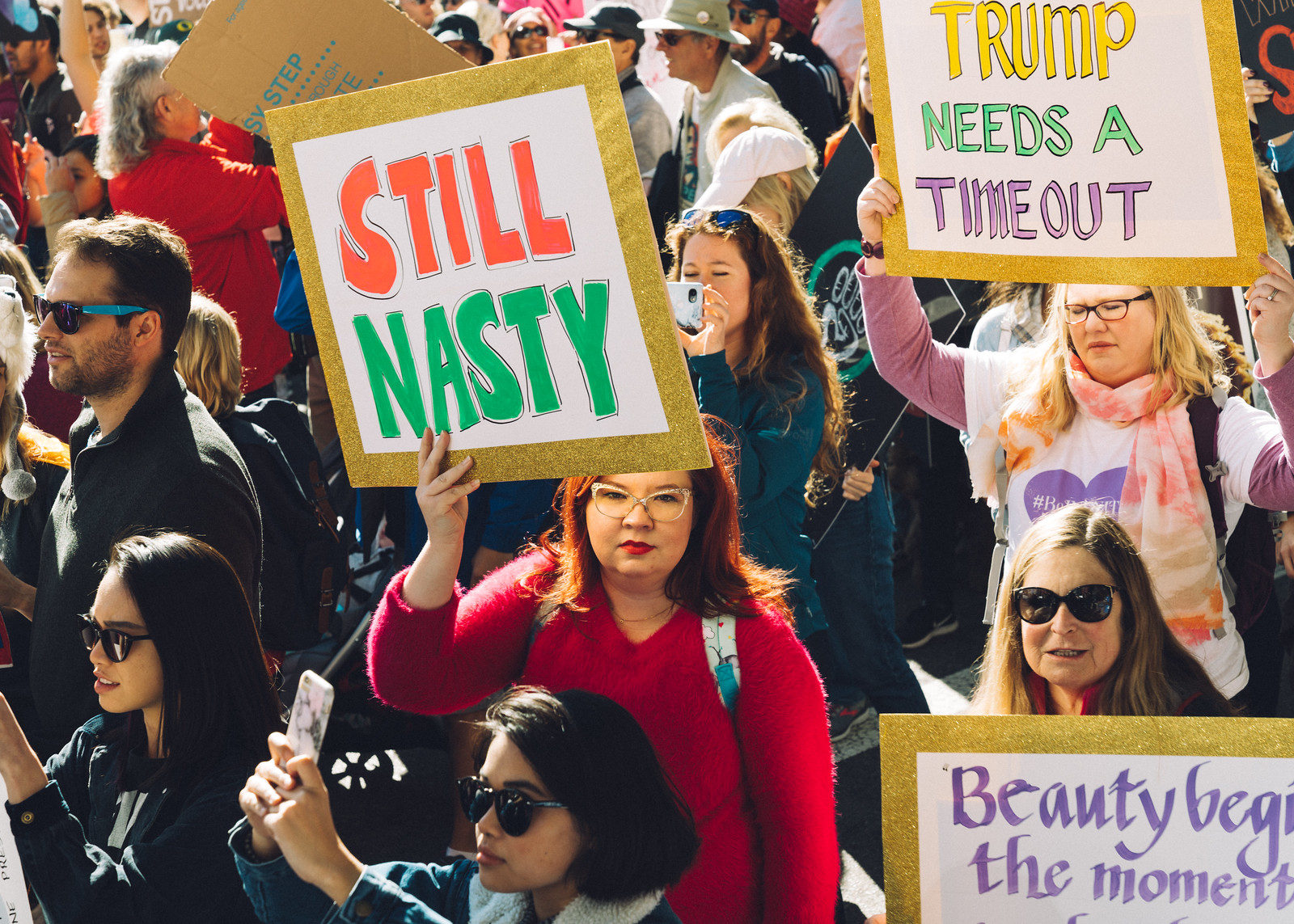In this horizontally aligned rectangular picture, a large, casually dressed crowd is gathered at a rally. Most people in the crowd are facing towards the left, but several individuals holding signs are facing directly towards the camera. At the center of the image stands a woman with reddish-brown, shoulder-length hair wearing eyeglasses and a long-sleeved red sweater. She is holding a square sign with a gold border and a white background that reads "Still Nasty," with "Still" in orange and "Nasty" in green, written in large, outlined letters. Behind her to the right, a blonde woman with glasses, clad in a white t-shirt and orange scarf, holds a similar sign with a gold border that reads "Trump Needs a Time Out," each word displayed in a different color. In the lower right corner of the image, another partially visible sign with a gold border reads "Beauty Begins the Moment," though the rest of the message is cut off. This lively snapshot appears to capture a diverse group of people, including a few men, attending a protest or rally, some holding signs, others holding phones.